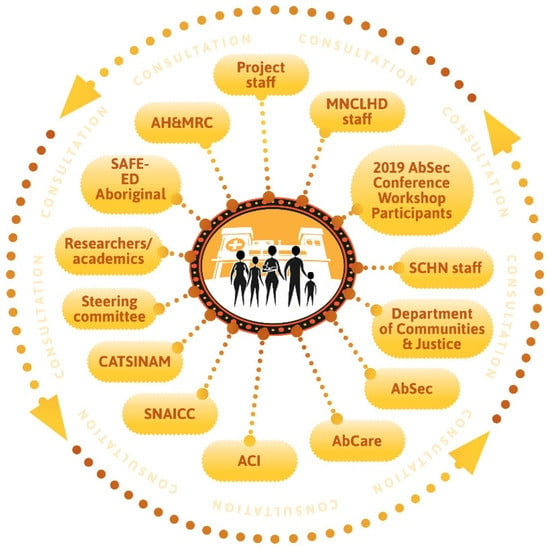The image is an intricate infographic designed in a circular layout, with a series of light brown, gold, and dark brown dots forming a detailed perimeter. This perimeter is bordered by four arrows positioned at intervals, creating a sense of movement around the circle, much like the hands of a clock. Along the interior of this circle, the word "consultation" is repeatedly inscribed in sloped letters, emphasizing the collaborative essence of the graphic.

At the core of the circle, there is an oval-shaped graphic featuring black, stylized silhouettes of a family comprising various figures — adults and children. This family stands in front of a building marked by a cross, indicating a medical facility or hospital.

Radiating from the central oval, black and gold dots branch out, forming connective stems to numerous labeled bubbles, each representing different groups or organizations involved in the project. These include "Project Staff," "CLHD Staff," "2019 ABSEC Conference Workshop Participants," "SCHN Staff," "Department of Communities and Justice," "ABSEC," "ACI," "SNAICC," "Katsunem," "Steering Committee," "Researchers and Academics," "Safe Ed Aboriginal," and "AH and MRC." These bubbles are depicted in either gold rectangles or ovals, emphasizing their importance and connection to the central theme of family and medical support.